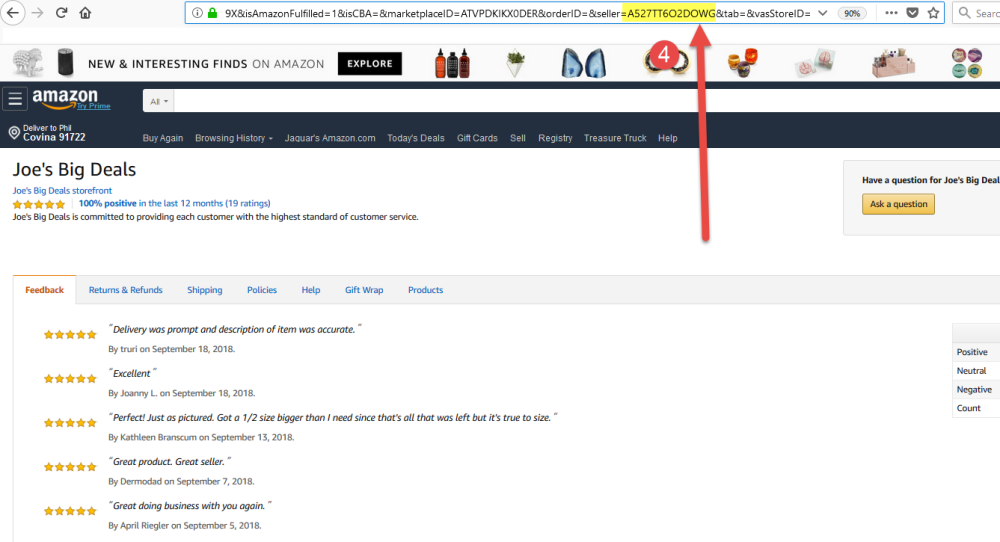This image shows the Amazon.com homepage, showcasing a variety of features and options for users. At the top, a banner reads "New and Interesting Finds on Amazon," with a clickable link to explore various items. Below this, the site features a search bar accompanied by quick links for suggestions, browsing history, buying again, today’s deals, gift cards, registry, Amazon’s Treasure Truck, and help.

Featured prominently is "Joe’s Big Deals" storefront, which has a high rating of five stars with 100% positive feedback in the last 12 months from 19 reviews. The store is committed to providing the highest standard of customer service. To the right, there is an option to ask questions directly to "Joe’s Big Deals". 

Further down, the page shows highlighted feedback, all rated five stars. Additional sections are visible for returns and refunds, shipping policies, gift wrapping, and product-specific information.